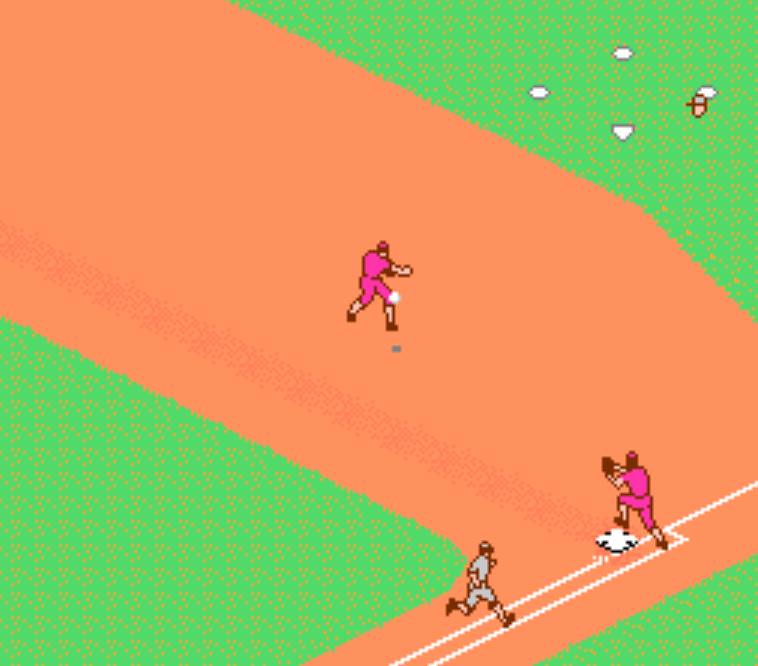This image is a screenshot from a baseball video game featuring a vibrant and detailed field. Predominantly, the scene is set against a backdrop of dark green grass dotted with patches of orange and light brown, giving the field a textured look. The gameplay shows three characters: two in bright pink uniforms and one in gray. Both pink-uniformed players, wearing matching hot pink caps and brown shoes, are positioned strategically on the field. One, standing on a white square base marked with four black dots at the corners, is ready with a dark chocolate-colored glove to catch the ball. The other pink player is mid-action, throwing a baseball, which casts a dark gray shadow on the ground. Meanwhile, the player in the gray uniform, also wearing a gray cap, is sprinting along white lines toward the base, trying to avoid being tagged out. The field is divided into sections: the vibrant green representing the grass, and large expanses of orange color with chocolate brown dots indicating the dirt areas. In the upper right corner of the image, four white dots, which likely denote direction, can be seen near the gray player's head.